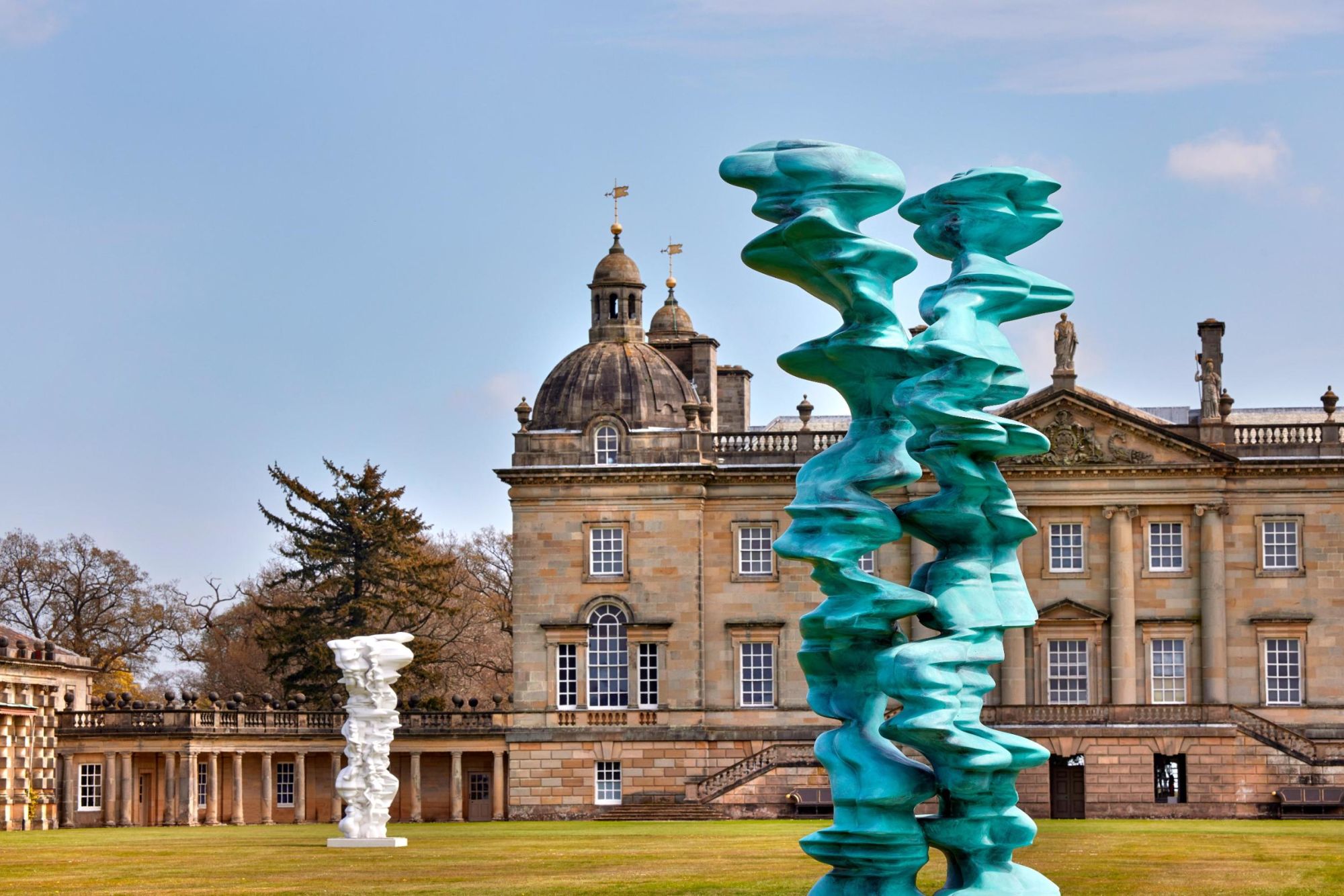This photograph captures the exterior of an old European manor, prominently featuring classic architectural elements such as columns, statues adorning the roof, and a stonework facade. The manor is a three-tiered structure with a small bell tower crowning its peak, and it is flanked by two domes bearing flags. Surrounding the manor is a meticulously maintained lawn, which serves as the setting for two distinctive sculptures. The foreground showcases a turquoise, abstract sculpture with a liquid-like, wavy form, reminiscent of eroded rock towers. A similar white sculpture stands in the distance, further enhancing the scene. Ornamental features such as a small fence on the roof and several spires add to the manor's grandeur. To the left, a staircase bordered by lush, evergreen trees and seasonally changing foliage leads up to the building. An auxiliary structure, slightly set apart, complements the main manor. The photograph, taken from the perspective of a sculpture garden, effectively combines the architectural beauty of the manor with the organic, flowing shapes of the sculptures, unified under a cyan-blue sky adorned with scattered clouds.